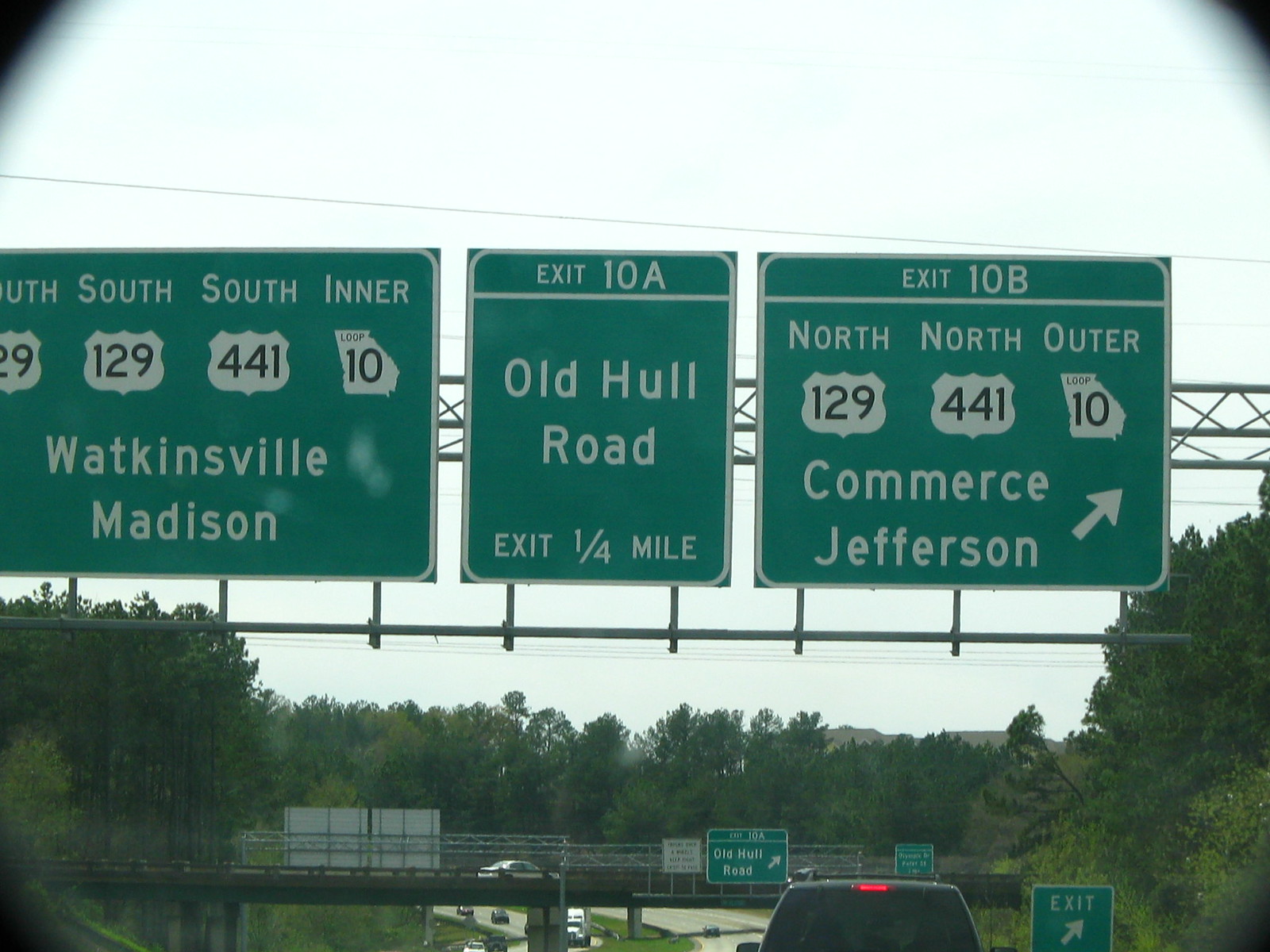The image depicts a set of three highway signs hanging above an interstate, positioned just above the middle of the frame. These signs are mounted on the usual metal grid structure seen on interstates. 

The first sign, slightly extending off the left side, displays directions for "South, Inner" with highway and interstate numbers 29, 129, 441, and 10. Beneath these numbers, the sign indicates the destinations "Watkinsville" and "Madison" in typical green and white coloring.

The middle, smaller sign provides information for exit 10A: "Old Hole Road, Exit 1/4 Mile." It is positioned directly to the right of the first sign.

The third and furthest sign to the right labels exit 10B: "North, South, Outer," along with highway numbers 129, 441, and 10. Below these, the destinations "Commerce" and "Jefferson" are listed, accompanied by a directional arrow.

At the very bottom of the frame, the top of a truck is visible. Beyond the vehicle, a bridge with grid railings can be seen, carrying another sign that repeats "Exit 10A, Old Hole Road." Immediately to the right of this is an indistinguishable green sign, a small white sign to its left, and another green sign reading "Exit" to the right of the truck. The scene is framed by a backdrop of trees on both sides and in the distance.